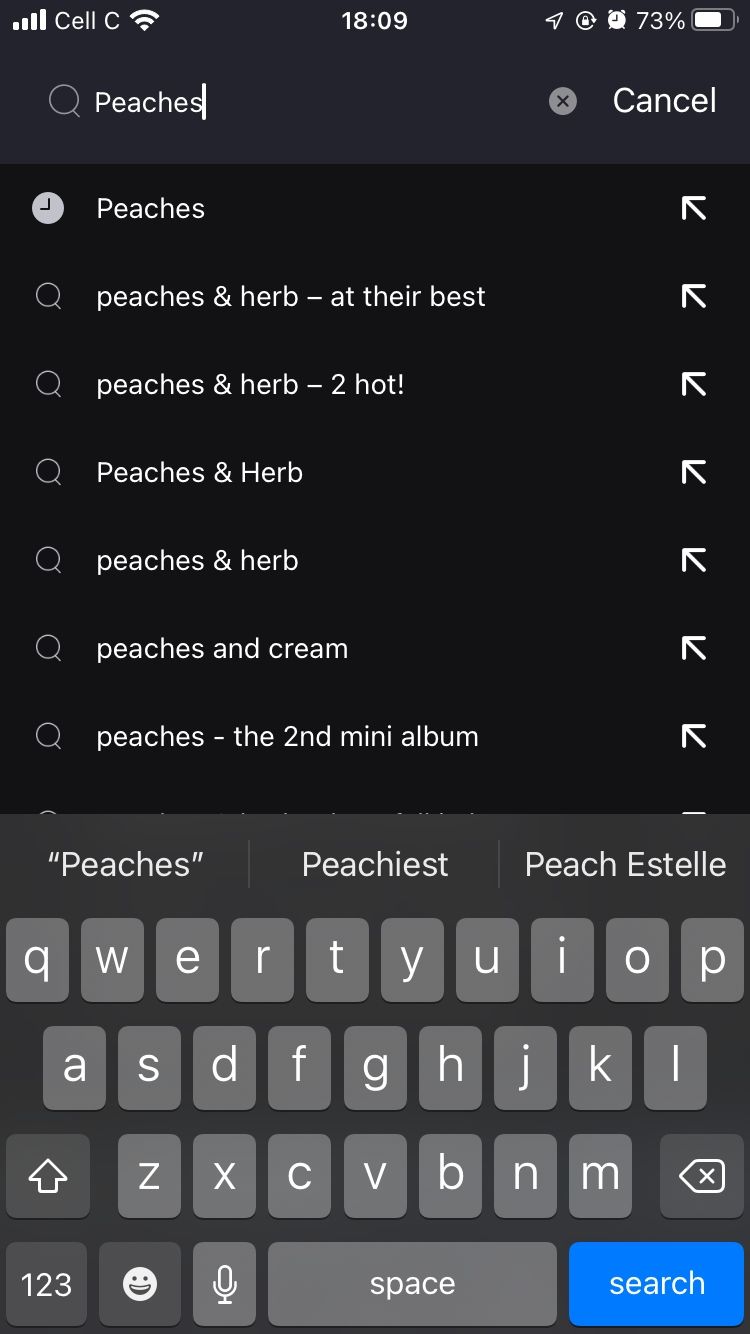The screenshot displays the interface of a mobile device, highlighting several on-screen elements and their functionalities. At the top, the signal status bar is visible, showing "Cell C," a signal strength indicator, a Wi-Fi icon, and the time "18:09." The battery icon displays "73%." 

In the content area, the screen has a black background with white text. The word "peaches" is written with a magnifying glass icon next to it, signifying a search bar. To the right, there is a gray "X" icon labeled "cancel."

Below the search bar, the list of search results is presented, each item with a white arrow on the left and a magnifying glass icon on the right. The list includes:
1. "Peaches & Herb at Their Best"
2. "Peaches & Herb Too Hot!"
3. "Peaches & Herb"
4. "Peaches & Herb" (repeated)
5. "Peaches and Cream"
6. "Peaches: The Second Mini Album"

Further down, suggested words appear in a predictive text area, showing terms like "peaches" (in quotation marks), "peachiest," and "peachestel."

At the bottom of the screen, there is a standard keyboard with a gray background and white letters. It features a numbers button, an emoji icon, a microphone button, and a blue and white "search" button. The fonts used are clear, bold, and easy to read, making the screen visually accessible. No additional objects or noteworthy items are present in the image.